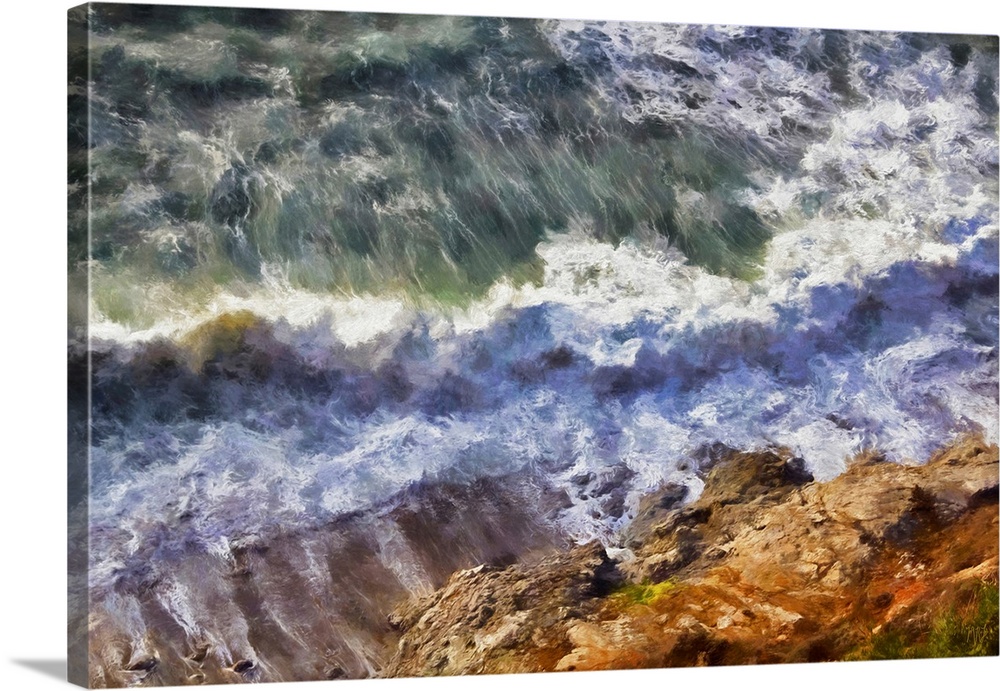This detailed image appears to be a decorative household painting, likely on a wrapped canvas, giving it a 3-dimensional appearance with visible borders on the left side. The scene depicted showcases a dynamic ocean landscape with vivid and expressive brush strokes. The bottom portion of the canvas features varying shades of brown, resembling rocky terrain interspersed with sand, complemented by hints of green to suggest vegetation. As the viewer's eye moves upwards, the rocks and sand transition into an animated ocean, where waves in shades of white and pale blue crash against each other. Within the middle segment, the waves become whiter and more turbulent, hinting at the shoreline. Further up into the top left, the colors shift to darker shades of blue and green, even approaching black, with splashes of white foam highlighting the restless sea. The top right is dominated by lighter colors, blending whites and subtle blues, creating contrast with the darker, more intense waves on the left. The overall composition captures the essence of a coastal scene, replete with the raw and natural beauty of crashing waves and rugged landscape.